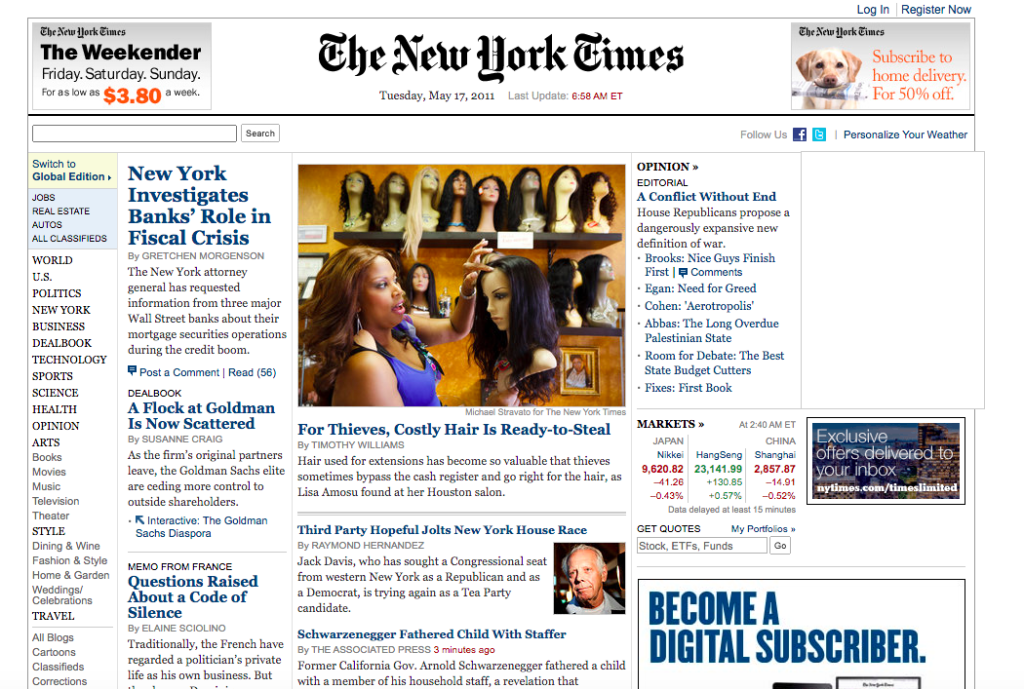Screenshot of a digital New York Times front page dated Tuesday, May 17th, 2011, last updated at 6:58 AM ET. The layout mirrors a traditional newspaper, with clickable article titles leading to full content. Each article appears with the title, author's name, and a brief introductory sentence. Below each blurb, there are options to post a comment and a note of the number of existing comments, denoted as (56). The header features options to log in or register, and a banner advertises a subscription deal: "Subscribe to home delivery for 50% off." An additional promotion in the upper left corner offers "The Weekender" package for Friday, Saturday, and Sunday deliveries at $3.80 per week.